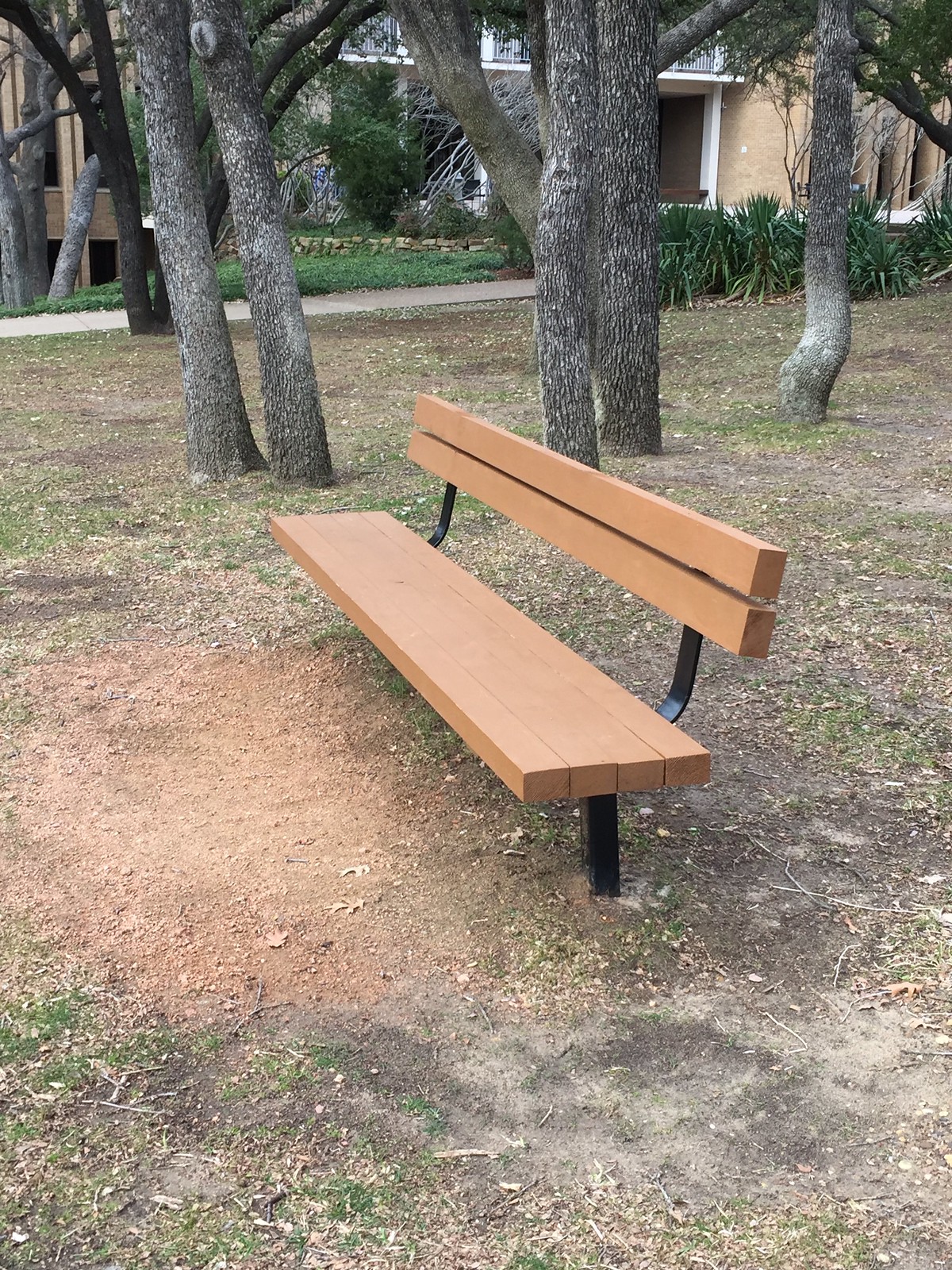This is a color photograph capturing a park bench situated in a wooded, park-like area with hints of an adjacent residential building. The bench is prominently displayed in the foreground, appearing new and made from medium brown wood with metal supports. The seat consists of four wooden slats, and the backrest of two angled wooden planks, all held together with sturdy black metal frames and posts, which are cemented into the ground to hold it in place.

The ground immediately in front of the bench shows patches of dirt and bare earth, indicating frequent use where feet have worn away the grass, leaving the surface reminiscent of the bench's brown color. Surrounding the bench, we observe an expanse of grass dotted with fallen leaves and small sticks, suggesting a seasonal shift toward autumn or winter.

In the background, several trees with grayish bark stand tall, their trunks adorned with remnants of limbs, characterized by distinctive circular marks. Further back from the trees, there is a notable presence of bushes and ornamental grasses. Beyond this greenery lies a large, light brown, possibly multi-story building with visible balconies, windows, and doors. This structure adds an architectural element to the natural scene, suggesting a residential area such as an apartment complex or housing unit.

Overall, this image portrays a harmonious blend of natural and man-made elements in an outdoor setting under an overcast sky, with a detailed foreground featuring the well-crafted bench and a rich background interspersed with trees and a residential building.